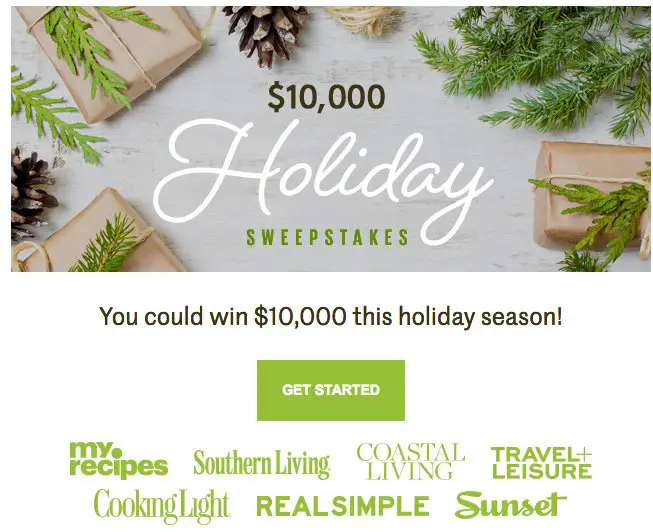The image portrays an assortment of parcels wrapped with twigs, branches, and pine cones, creating a rustic, festive atmosphere. At the center of the rectangular picture, a prominent "$10,000" is displayed in brown lettering. Below this, in large white font, the word "HOLIDAY" is prominently featured. Directly beneath, in bold green capital letters, the word "SWEEPSTAKES" stands out, forming the phrase "10,000 HOLIDAY SWEEPSTAKES". 

Underneath this header, a sentence in brown reads, "You could win $10,000 this holiday season!". Below this enticing message is a green button with the text "Get Started" in white lettering. 

Further down, a collection of seven brand names is presented. Starting from left to right in the first row are: MyRecipes (capital 'M' and 'R'), Southern Living (capital 'S' and 'L'), and COASTAL LIVING (entirely capitalized). Next, "TRAVEL + LEISURE" appears, fully capitalized on the same row. On a new line below, the brands Cooking Light (capital 'C' and 'L'), REAL SIMPLE (entirely capitalized), and Sunset (capital 'S'), complete the list. 

This image brings together the elements of holiday cheer and the excitement of a potential $10,000 win, emphasizing the joyous and lucrative possibilities of the season.